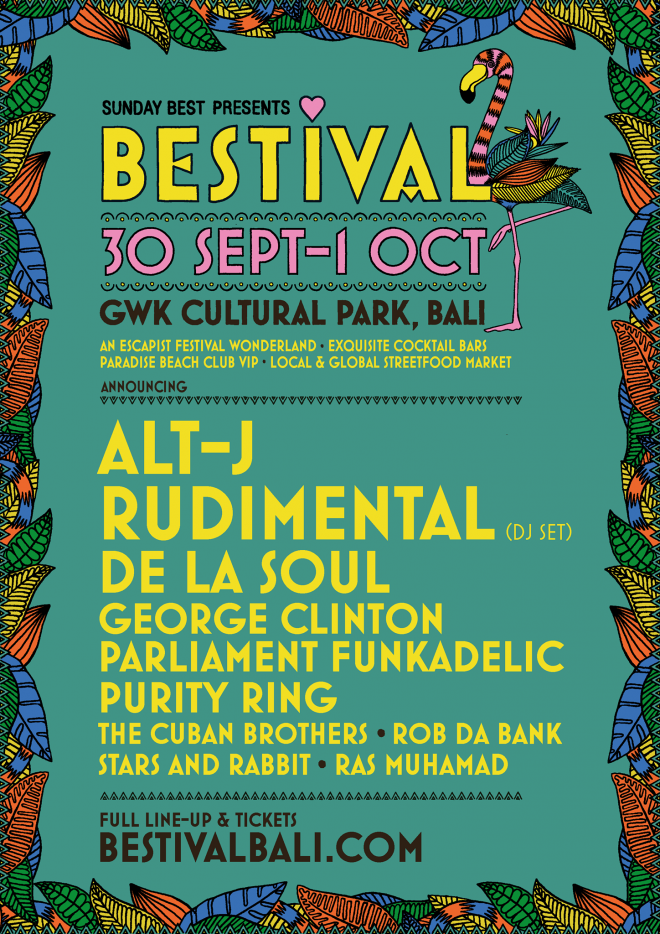This vibrant advertisement features a blue background adorned with various tropical leaves in shades of orange, yellow, and green, creating a lively border around the long rectangular layout. At the top, it reads "Sunday Best Presents" followed by a pink heart symbol. Below that is the word "Bestiful," interrupted by an illustration of a flamingo with a striped neck, leafy body, long yellow beak with a black tip, seamlessly integrated into the text. To the left of the flamingo, the dates "30th September – 1st October" are highlighted in pink. Beneath it, "GWK Cultural Park, Bali" is prominently displayed. Further down, in yellow text, enticing details include "Escape Festival Wonderland," "Exquisite Cocktail Bars," "Paradise Beach Club VIP," and "Local and Global Street Food." The lineup announcement follows in yellow, listing artists: Alt-J, Rudimental, De La Soul, George Clinton & Parliament-Funkadelic, Purity Ring, The Cuban Brothers, Rob Da Bank, Stars and Rabbit, and Ras Mohammed. For more information and tickets, the text directs visitors to "BestifulBali.com."